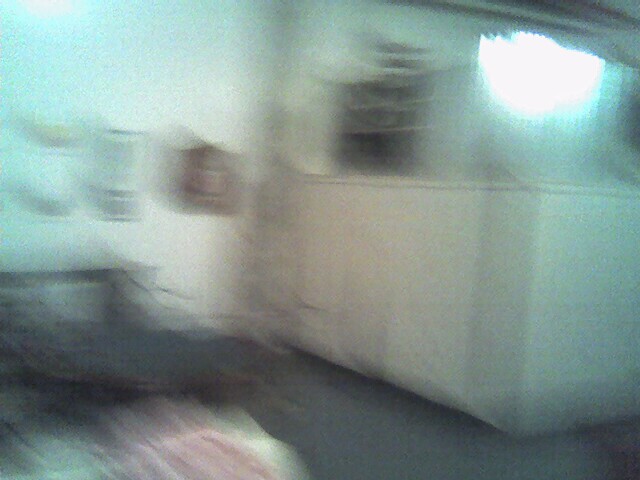The image depicts an out-of-focus, heavily blurred indoor scene with dominant blue-green coloring. The setting appears to be an office environment due to the presence of what might be a cubicle with white walls and a potential white partition. On the left side, there is a suggestion of a dark doorway or window, while near the center, there is either a large white container or bin. Above the partition, a large beam of bright light, possibly from a window, illuminates the area. The floor appears blue with hints of brown areas, which might suggest a carpet or flooring with mixed colors. There are some unidentifiable rectangular shapes and faint pink and green hues on the ground. The wall, spanning from floor to ceiling, has several indistinct images or flyers hanging, and a blurry brown, possibly wooden, object - maybe an armoire or shelf - is partially visible, adding to the room's office-like atmosphere.